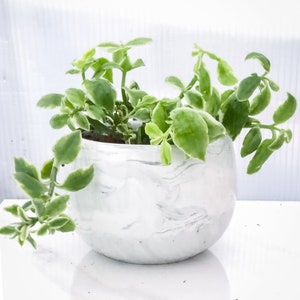In this bright and artistic photograph, a delicate house plant with soft, green, leaf-shaped leaves edged in white is the focal point. The plant, which resembles a vine or ivy, has one elegant tendril cascading over the side of its container, reaching down toward the shiny white tabletop below. The plant is potted in a beautifully simple, rounded, white porcelain planter adorned with subtle streaks of gray, giving it a sophisticated yet understated appearance. The backdrop is a muted grayish-white wall, adding to the minimalistic and serene composition. The image is predominantly white and green, capturing a serene and stylish aesthetic often seen in elegant home décor or coffee table books.